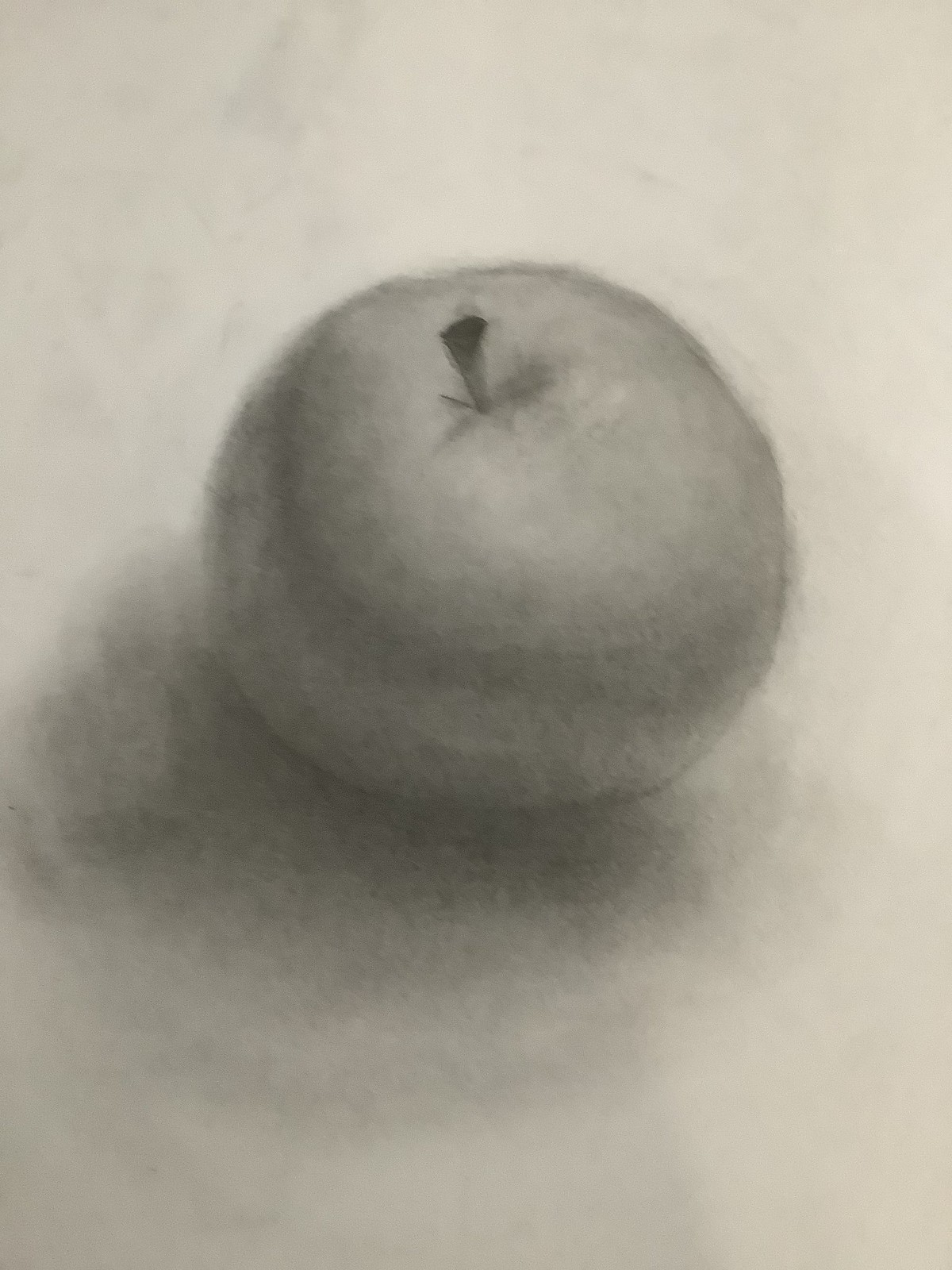The image portrays a penciled sketch of an apple, centered on a white page, drawn primarily with pencil and possibly some charcoal or chalk. The Apple itself has an orb-like shape with notable shading on the left and front, suggesting a light source from the upper right. The apple is topped with a small stem extending straight up. The overall drawing emphasizes shadowing beneath the apple and in the lower left, creating a sense of depth. The image is somewhat out-of-focus, which contributes to a lack of sharpness and detail. The background remains predominantly white with minimal shading in the lower right section. The drawing is unsigned, without any text or additional markings. Despite the simplicity and lack of vibrant colors, this sketch stands out as a well-executed study of an apple.